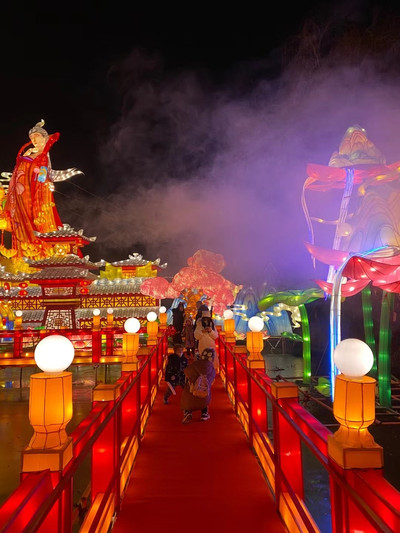This image, taken during the Chinese Lantern Festival, also known as the Mid-Autumn Festival, showcases a family scene set against an intricately designed and brightly lit walkway. The family, consisting of a few adults and children, walks along a red carpeted path that serves as a bridge over water, enclosed by red and orange walls. Along the top of these walls, yellow lanterns with circular white globes illuminate the scene.

The nighttime setting is enhanced by a misty fog, adding an ethereal quality to the photo. On the left side, a vibrant red and yellow-orange figure of a woman, constructed from materials resembling tissue paper and lit up like a parade float, commands attention. Opposite her, a series of neon-lit trees feature brilliant green bamboo trunks with red flowers. The backdrop reveals traditional Chinese architecture with multi-layered, colorful facades that suggest a festive atmosphere.

Dominant colors include gold, red, green, and blue, creating a vivid and celebratory ambiance appropriate for the Festival, emphasizing the tradition and imagination characteristic of such an event.